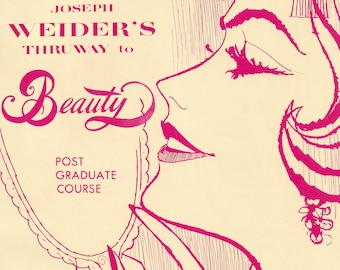The image is an old-style advertisement, likely from the 1920s or 1930s, illustrated in a retro style on a white paper background with black ink and a pinkish hue. Dominating the right half of the image is a glamorous woman, whose profile reveals only the left side of her face. She has short hair, a tiny mole above her lips, and is adorned with dangling earrings. Her face is beautifully made up with lipstick, mascara, and distinct eyebrows, all contributing to her elegant, smiling expression. The woman appears to be gazing into her reflection in a handheld mirror situated on the left side of the image. In the upper left corner, the text reads "Joseph Widener's Way to Beauty," followed by "Postgraduate Course" in smaller text below. The overall composition strongly evokes a vintage beauty advertisement.